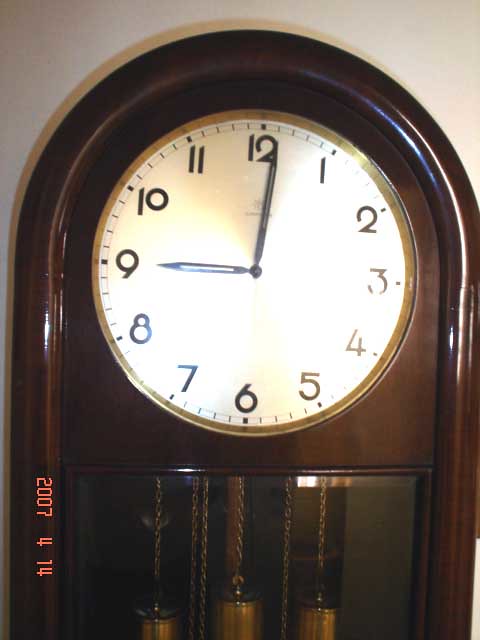This image captures a close-up of a large, traditional grandfather clock, showcasing its elegant and intricate details. The clock features a polished, dark wood frame with a reflective finish and an arch at the top. The clock face, situated just beneath the arch, has a white background with a gold trim, black numerals from 1 to 12, and black hands indicating the time as 9:01. There is a double ring marking the minutes along the clock's edge. Below the clock face, the polished wooden frame continues and leads to a glass panel. Inside the glass, one can see three weights suspended on gold chains, suggesting the pendulum mechanism. The image is dated with a timestamp in pink letters reading "2007-04-14." The clock's grandeur is evident, although the full length of the clock is not visible in the photo.